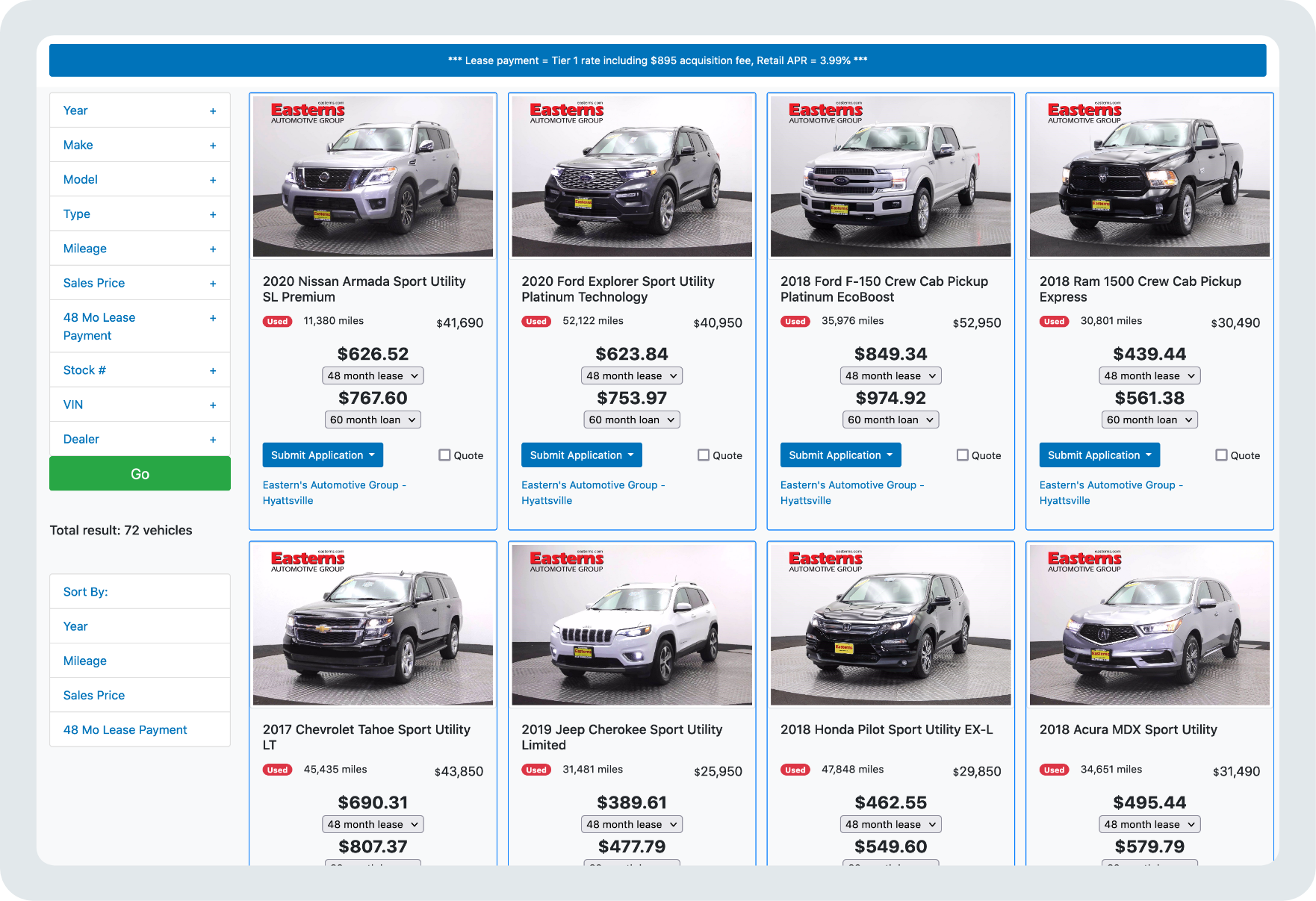This detailed image showcases a comprehensive overview of various vehicles available for lease, including specific financial and identification information. At the top, lease payment details are prominently displayed, highlighting a Tier 1 rate that includes an $895 acquisition fee with a retail interest of 3.99%. The left pane of the image systematically presents the essential attributes of each vehicle, such as the year, make, model, type, mileage, sales price, 48-month lease payment, stock number, and vehicle inspection number.

The image features a total of 72 vehicles, which include notable models such as:
- 2020 Nissan Armada, Armada Sport Utility, SL Premium
- 2020 Ford Explorer Sport Utility
- 2018 Ford F-150
- 2018 RAM 1500 Crew Cab Pickup
- 2018 Acura MDX

This detailed layout helps in understanding the leasing options and specifics of each vehicle clearly, thereby aiding potential lessees in making informed decisions.